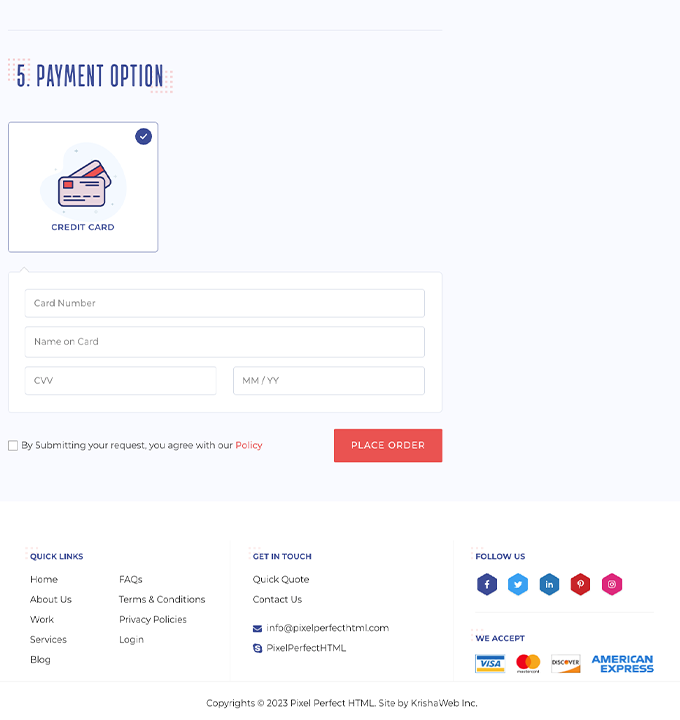The screenshot depicts a payment information page with several distinct elements meticulously arranged for user convenience. 

At the top left, the header "Payment Option 5." is displayed in a slightly bolded navy blue font. Adjacent to this text, there are several small orange dots arranged diagonally, adding a distinctive design touch.

Directly below this header is a light gray box with a white background containing an image of stacked front and back views of a credit card. The box is labeled “Credit Card”. Within this section, users are prompted to enter their credit card information, including fields for the credit card number, the name on the card, and two smaller fields for the CVV and the card's expiration date (MM/YY format).

Below the credit card information fields, there is a checkbox accompanied by a statement that reads, "By submitting your request you agree with our policy."

At the center of the page, there's a prominently displayed coral-colored button labeled "Place Order."

The bottom section of the page comprises quick links for easy navigation, including "Home," "About Us," "Work," "Services," "Blog," "FAQs," "Terms and Conditions," "Privacy Policy," and "Login." 

Additionally, contact information is provided under the "Get in Touch" section, listing the company's name (QuickCode), website, Skype, and email details. Social media follow buttons and icons representing accepted payment types are also present, ensuring users have all necessary details for transactions and further interaction with the service.